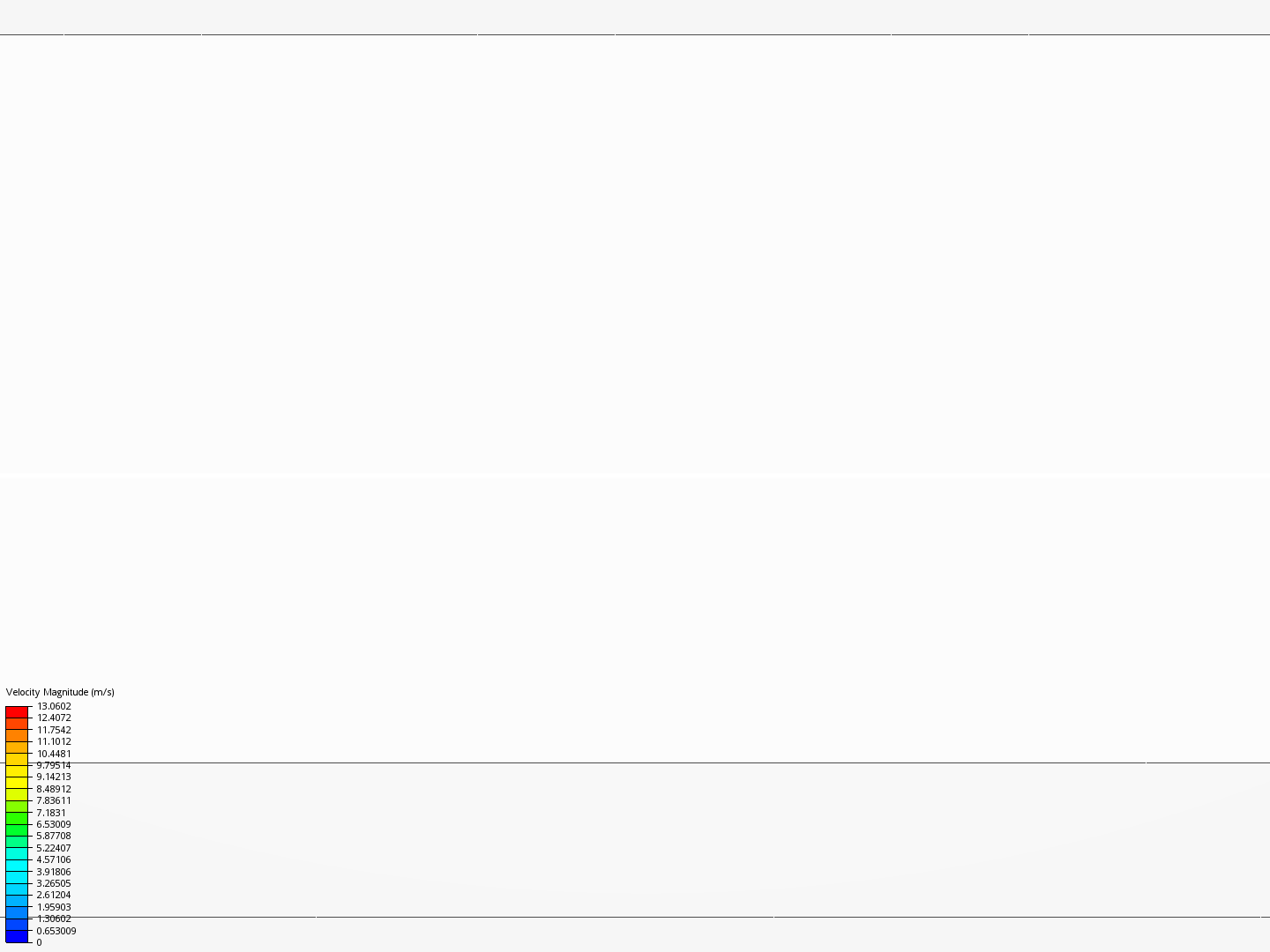The image depicts a computer screen displaying a graphical representation of velocity magnitudes. The screen is divided into three distinct regions: the top and bottom sections are shaded in gray, while the central section is white. 

On the left-hand side of the image, there is a vertical color scale labeled "Velocity Magnitude (m/s)." This scale showcases a gradient of colors that represent different velocity values. At the top of the scale, the highest velocity, indicated as 13.0602 m/s, is marked in red. As the velocity values decrease, the colors transition smoothly through a spectrum: from red to reddish orange, orange, orangish yellow, golden yellow, yellow, greenish yellow, green, greenish blue, blue, and finally reaching a deep royal blue at the bottom. Corresponding velocity values range from 13.0602 m/s at the top to 0 m/s at the bottom.